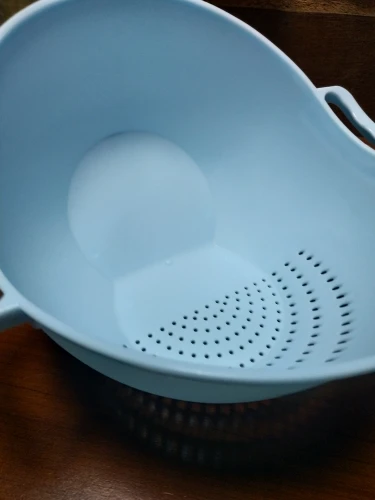The image features a light sky-blue, oval-shaped colander made of plastic. The colander has a unique design with holes covering about a third of one side, arranged in a semi-circular pattern to facilitate drainage. The device has thin walls and is equipped with small handles on both sides, although only the right handle is fully visible, with the left one being partially cut off. The colander is resting on a brown, wooden table, which serves as the background for the image.